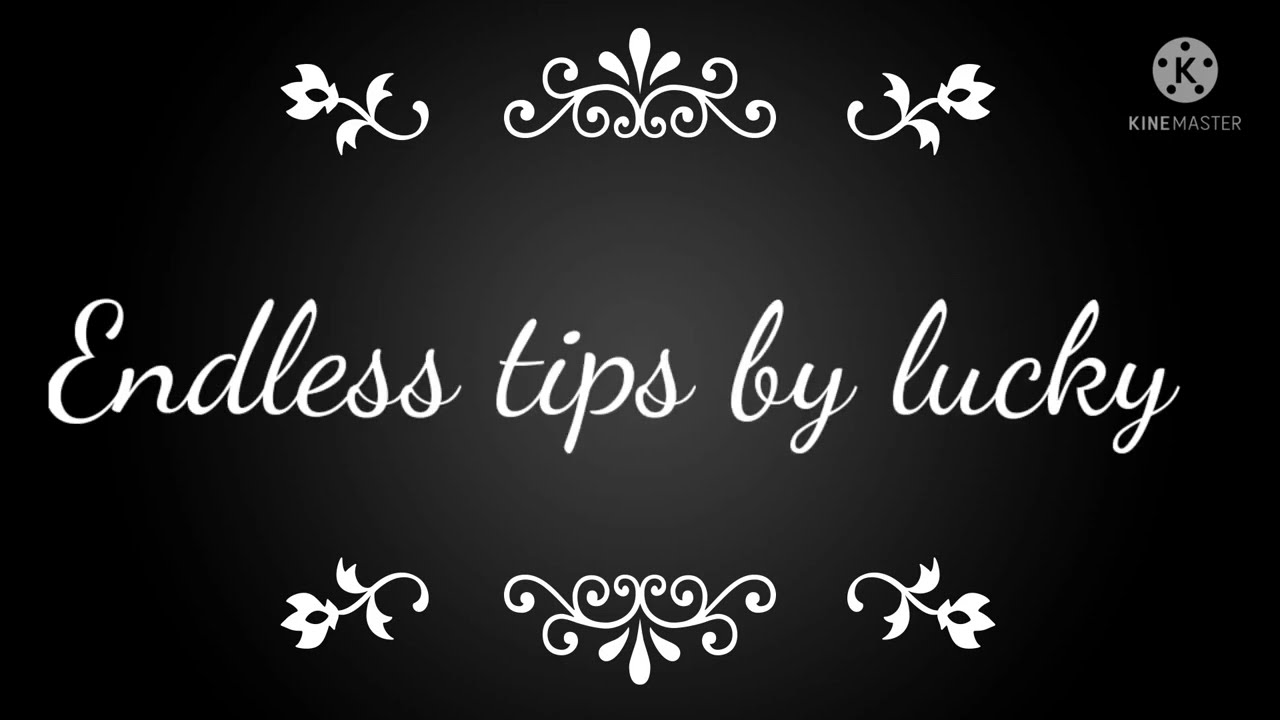The image is a glossy, black rectangle featuring a decorative card or placard. At the top right corner, a white circular logo with a capital “K” in the center is surrounded by five smaller black dots arranged in the pattern of a star, with "KineMaster" inscribed beneath it. In the center of the image, spanning the horizontal middle, is the phrase "Endless Tips by Lucky" written in elegant white cursive script. The top and bottom of the card are adorned with symmetrical, ornate designs. These designs consist of a central flowery vine with three petals, flanked on each side by a flower with leaves and stems, mirroring each other: the top design points outward, while the bottom design is inverted, pointing inward.